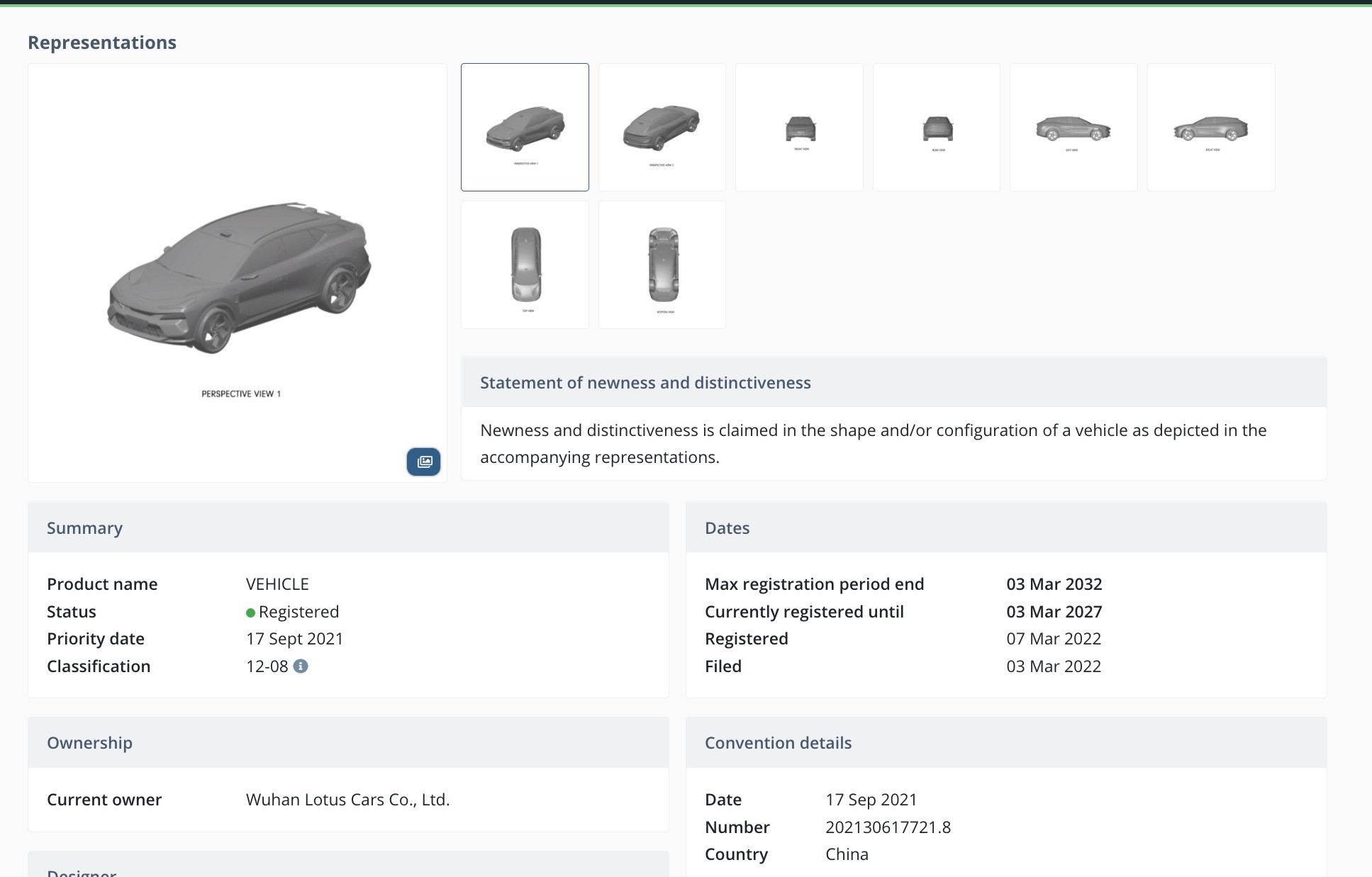This image depicts a web page displayed on a PC screen. The top of the page features a narrow black line running horizontally across its entire width. Just beneath this line, the word "Representations" appears aligned to the left. Below this section is a series of grayscale illustrations of a car, showcasing different perspectives and angles. The illustrations include views from the front, driver's side, back-from-the-driver’s-side, back-from-the-passenger’s-side, rear, front again, side, another side straight on, and a top view. 

Further down, the text "Statement of Newness and Distinctiveness" is prominently displayed. Under this heading, starting from the left, is the section labeled "Summary," highlighted in a gray bar extending to the middle of the page. Adjacent to it, the gray bar continues across the page with the heading "Dates." Beneath these headings, the page lists various details in black text against a white background. The details include: Product Name, Status, Priority Date, Classification, Ownership, Current Owner, Maximum Registration Period, and Currently Registered Until. Each of these sections features its own gray bar header that spans horizontally across the page. The overall layout is clean and text-focused, designed for clarity with consistent gray bar headings and black text on a white background.